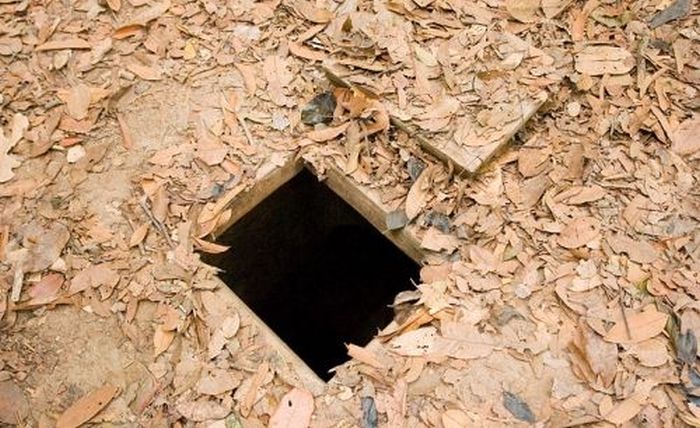This image showcases an outdoor scene dominated by a bed of brown and orangish leaves, indicative of fall. The ground is strewn with leaves, creating a natural camouflage for the central feature of the photograph: a black, square hole. This hole, slightly off-center towards the bottom left, appears to be man-made with wooden edges rather than a naturally occurring depression in the earth. The opening looks deep and dark, its bottom obscured from view. Positioned towards the top right, partially covered by leaves, is a wooden square lid designed to fit securely over the hole, suggesting it is a concealed or hidden entrance to something underground, possibly a well or storage area. The setting lacks any text and features a palette primarily consisting of various shades of brown, tan, and black, reinforcing the natural and somewhat mysterious atmosphere of the photograph.